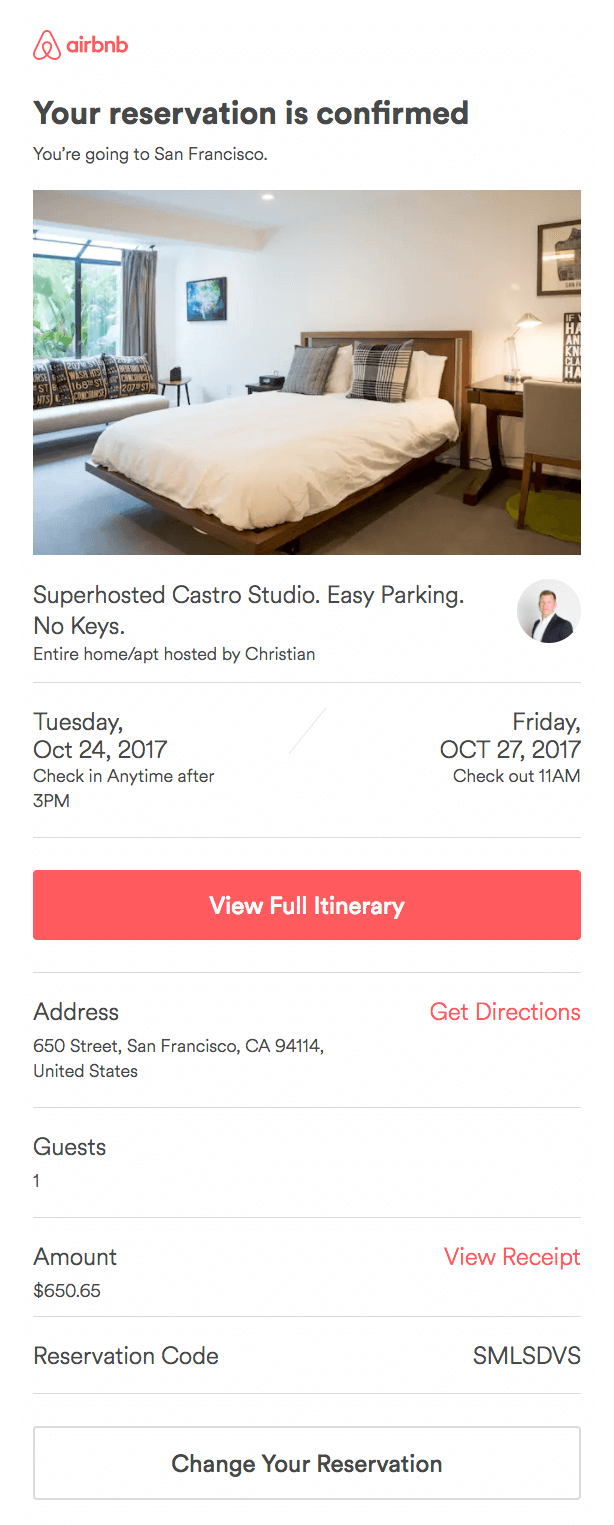**Airbnb Reservation Confirmation for San Francisco Trip**

At the top of the image, the iconic Airbnb logo is prominently displayed, resembling a red arrow with intricate curls in the center, alongside the text "Airbnb" in bold lettering. Below the logo, a bold black heading announces, "Your Reservation is Confirmed." Further down in black text, it cheerfully states, "You are going to San Francisco."

The image showcases a cozy bedroom. On the left, a large window illuminates the room with natural light. The bed, prominently positioned, features a flat structure with a pristine white sheet. To the right of the bed, a wooden nightstand complements the wooden frame of the bed. Black cushions with gold and brown accents add a touch of elegance. The room's floor is covered with short dark gray carpeting, and the walls are painted a clean white.

Beneath the bedroom image, black text highlights the details: "Super Hosted, Castro Studio, Easy Parking, No Keys." It describes the accommodation as "Entire Home/Apt hosted by Christian." To the right, a circular portrait shows the host, Christian, with short brown hair, light skin, wearing a white dress shirt and a black tuxedo against a dark gray backdrop.

Further details include:
- **Reservation Dates:** Tuesday, October 24th, 2027, to Friday, October 27th, 2027.
- **Check-in Time:** Any time after 3 p.m. on October 24th.
- **Check-out Time:** 11 a.m. on October 27th.
- A red clickable button with white text says, "View Full Itinerary."

Address details are provided with the location: "650 Street, San Francisco, CA 94114, United States." There is a hyperlinked "Get Directions" in red text.

The reservation summary lists:
- **Guest Count:** 1
- **Amount Due:** $650.65
- **Reservation Code:** SMLSDBS

Final actions are facilitated with a clickable red button reading, "Change Your Reservation," at the bottom of the image.